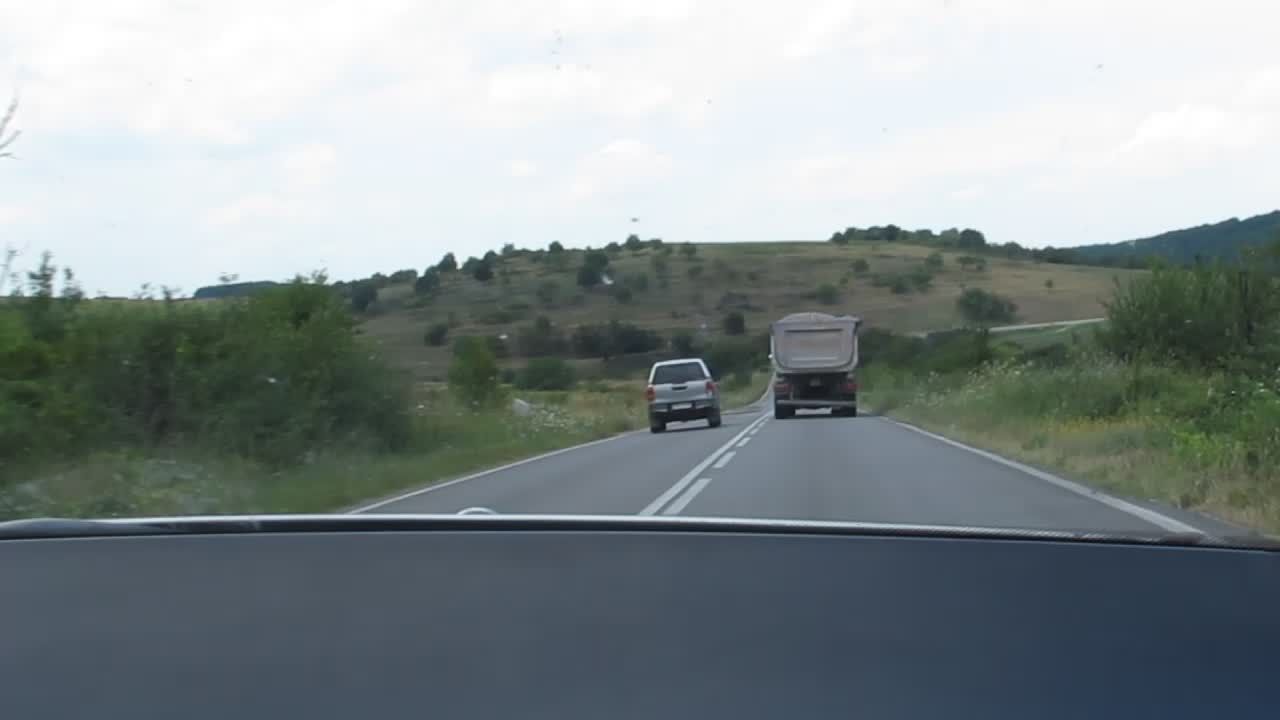A desaturated, horizontally-framed color photograph captures a scene from the front of a car on a typical two-lane road. The image features two vehicles ahead, a large truck and a smaller car, both traveling in the same direction. Beyond the road, a backdrop of distant mountains can be seen under an overcast, white sky. The muted tones of the image evoke a subdued, almost melancholic atmosphere.